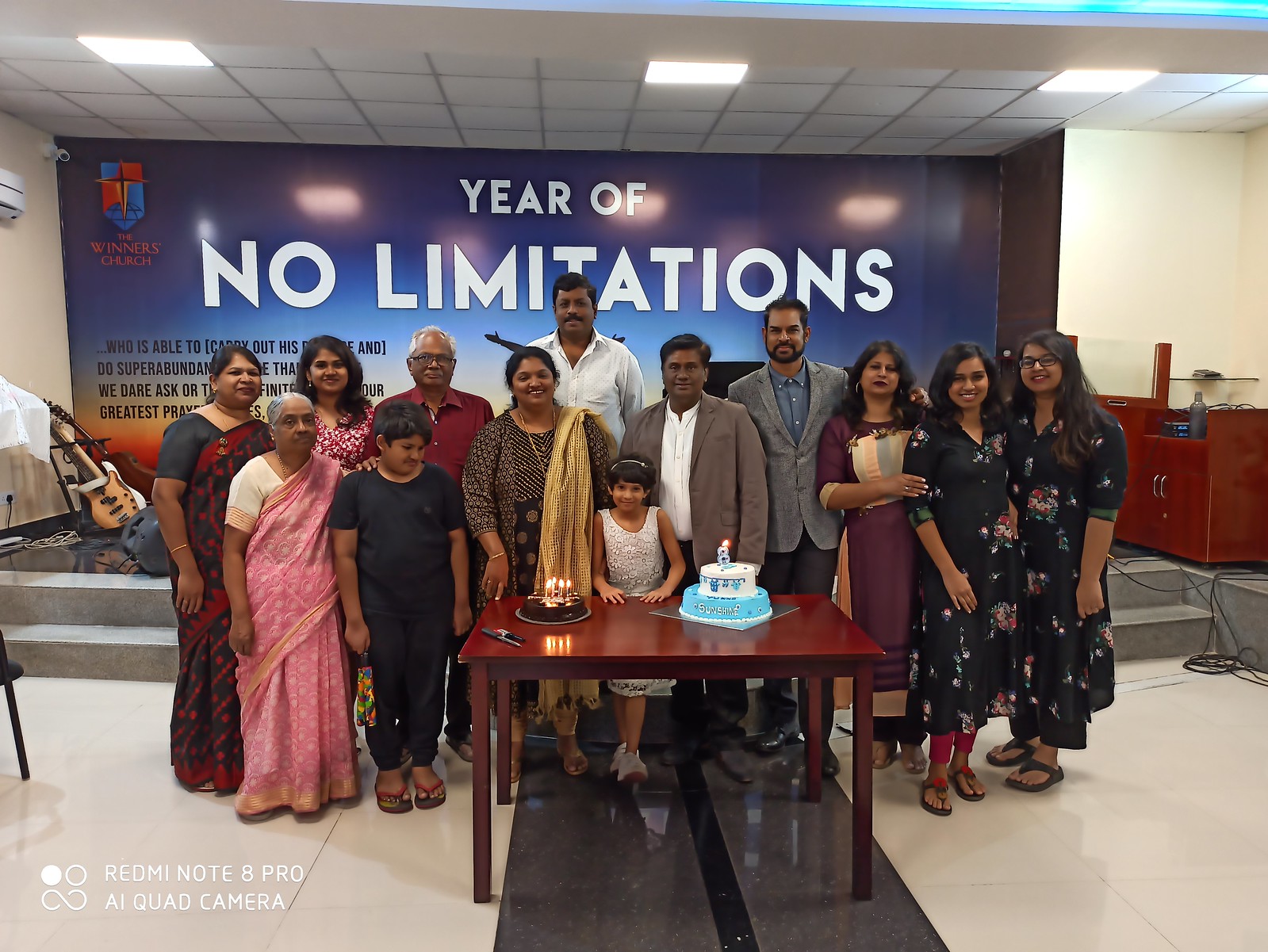The image captures an indoor celebration, likely a family birthday party, prominently featuring a diverse group of 13 people ranging from young children to older adults, who appear to be of Indian descent. The group is posing around a wooden table set on a white tile floor with gray details. On the table are two cakes: a blue and white cake on the right with an "8" candle and a chocolate cake on the left adorned with several lit birthday candles. At the center front, a smiling little girl stands out in the group. The background shows a white tile ceiling and a banner that reads "Year of No Limitations" in white on a blue backdrop. Additional details include a stage with musical instruments and a logo with a cross with the text "The Winners Church." At the bottom of the image, the text "Redmi Note H Pro AI Quad Camera" is visible.